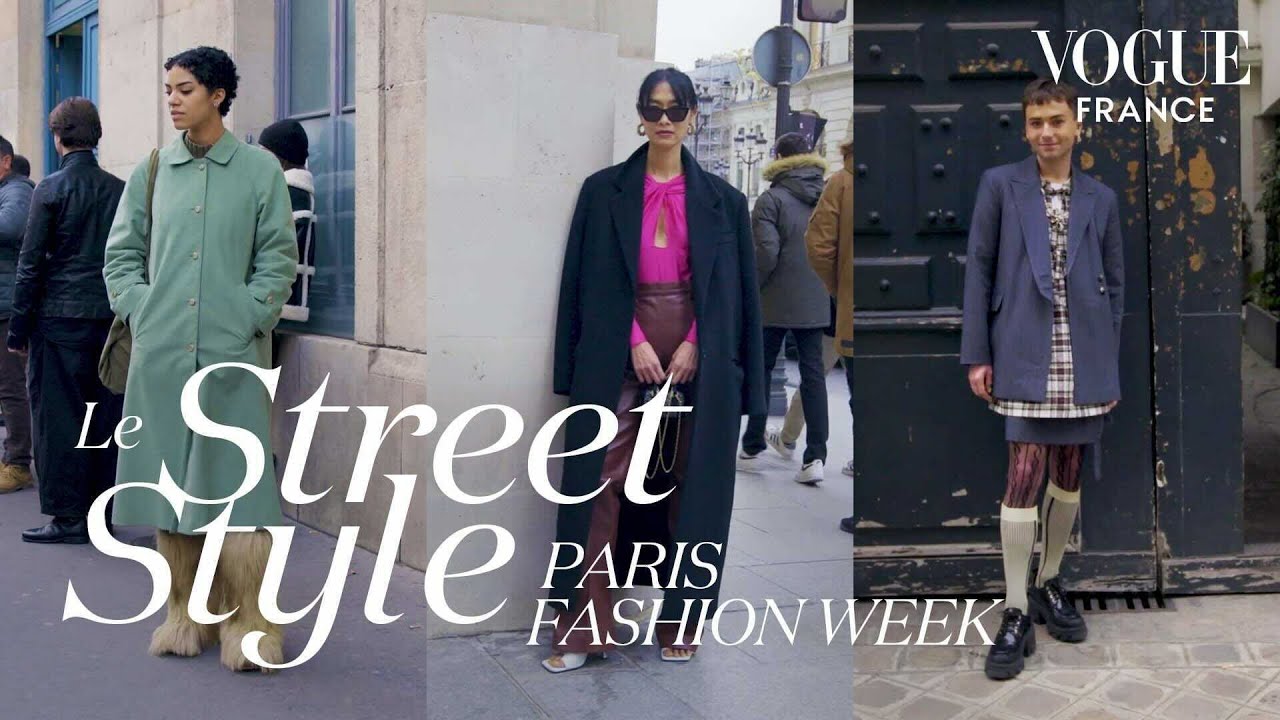The image features a promotional collage for Vogue France, highlighting street style at Paris Fashion Week. There are three distinct photographs arranged side by side, each showcasing different fashion-forward individuals. 

On the left, a light-skinned black woman with short, curly hair dons a long sage green trench coat that extends to her shins. She completes her outfit with fluffy cream-colored boots reminiscent of Chewbacca's fur, and carries a purse. 

In the center, a woman is seen wearing an eye-catching ensemble consisting of a pink top, dark red leather pants, and white sandals. She adds a touch of sophistication with a long, flowing navy blue trench coat left open, and accessorizes with dark black sunglasses and her short black hair styled sleekly to the side.

The right image displays a man dressed in a fashion-forward combination of a navy blue coat over a patterned white shirt. He pairs this with a short blue skirt, burgundy plaid tights over white stockings, and black platform boots. 

The setting is brightly lit, ensuring each colorful outfit and detail stands out clearly. The top right corner bears the Vogue France logo, while the bottom center of the collage reads "La Street Style Paris Fashion Week", emphasizing the chic and diverse street styles captured at the event.